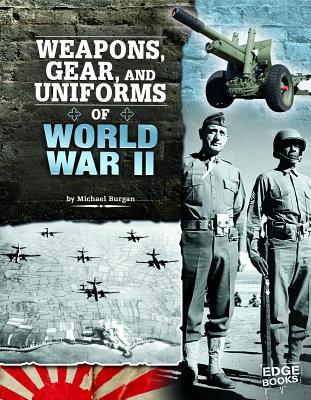The image depicts a detailed book cover, likely a historical reference guide titled, "Weapons, Gear, and Uniforms of World War II," authored by Michael Bergen. The book cover is primarily in black and white with distinct colored elements, creating a visually segmented layout. The upper left corner features a dark, almost black, brick wall background with bold white text listing the title, while the words "World War II" appear in light blue. Beneath this, a lighter gray landscape portrays Japanese planes flying, symbolizing the era's military aviation. The iconic red and white Rising Sun flag of Japan is situated at the bottom center of the cover. On the right side of the cover, a composite image displays a World War II military scene: a cannon on a wheeled chassis aims leftward above two soldiers standing at attention. The soldier on the left, an officer in a peaked cap, wears a detailed combat belt and a full military uniform, while the soldier on the right, donning a helmet, holds a rifle with its muzzle resting on the ground. Both soldiers are depicted in authentic 1940s military attire. The lower right corner prominently features the Edge Books logo in bold white lettering, contributing to the historical and authoritative aura of the cover.